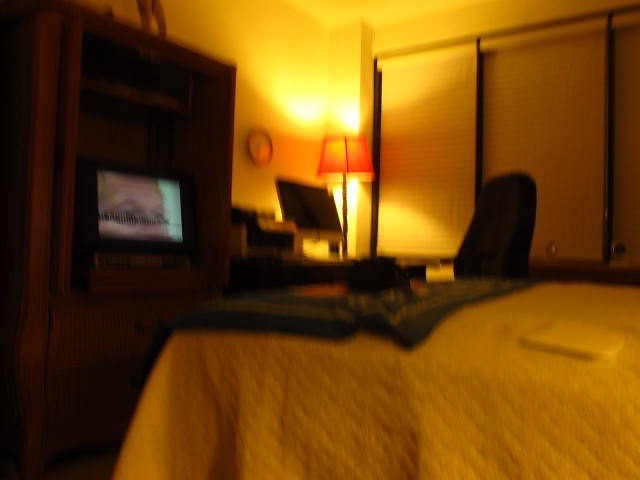The image depicts a warmly lit, yellow-hued room interior. In the bottom-right portion, there is a bed adorned with a white bed cover, a book resting on the right side. Draped over the front of the bed to the left is a green cover with some black items placed atop it. On the left side of the image stands a brown, wooden cabinet housing a TV with black bezels, displaying some content. Toward the top of the image, a black chair is positioned in front of a table situated in the corner. The table hosts a computer screen, characterized by a silver bezel and a black display. Illuminating the scene, a yellow-hued light gleams, while a circular analog clock is mounted on the wall. Additionally, there are blinds located on the upper part of the room, specifically in the top-right section of the image.